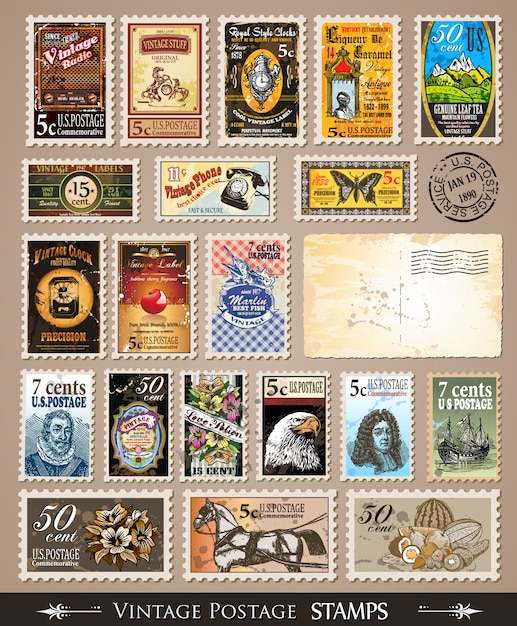The image is a portrait-oriented poster showcasing a grid of vintage postage stamps, labeled with "Vintage Postage Stamps" in white text at the bottom against a black border. The stamps are not perfectly arranged but are presented in five distinct rows. Highlights include a variety of stamps, such as an 11 cent vintage phone stamp labeled "Best choice ever. Fast and secure," a 7 cent U.S. postage stamp featuring a ship, and a 5 cent U.S. postage stamp with a horse hooked to a wagon. Among other captivating stamps, there's a 50 cent stamp with fruit, a vintage clock stamp marked "precision," a 5 cent stamp with a vintage radio, a U.S. postage stamp with an American eagle, and a celebratory stamp from January 19th, 1890, capturing a snapshot of historical postal services. The overall background of the image is a dark grayish-brown, enhancing the nostalgic feel of this meticulously curated stamp collage.